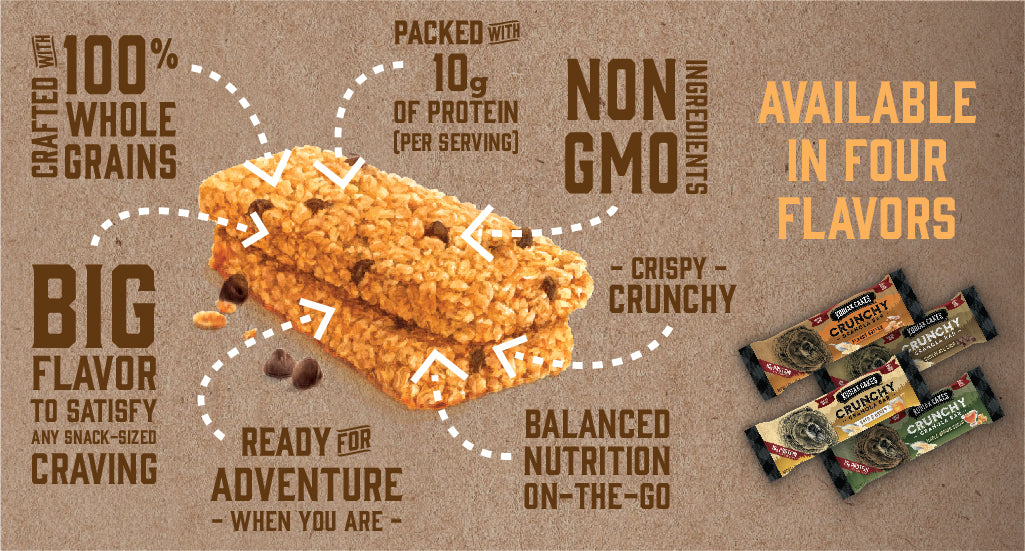This advertisement features a selection of four crunchy granola bars prominently displayed on the right side, each wrapped in distinctively colored packaging—orange, tan, gold, and green. The packages are all emblazoned with the word "crunchy" and an illustration of a grizzly bear's face roaring towards the viewer. The two unwrapped bars in the center are stacked, showcasing their texture packed with chocolate chips and possibly peanuts, with additional chocolate chips scattered around them.

The background gives an earthy, rustic feel with an unbleached paper effect, further enhancing the natural appeal of the product. Surrounding the granola bars are several descriptive text elements in brown, connected by dotted arrows. These text highlights emphasize the product’s key features: crafted with 100% whole grains, non-GMO ingredients, packed with 10 grams of protein per serving, crispy and crunchy texture, balanced nutrition on the go, and big flavor to satisfy any snack-size craving. It also carries motivational slogans like "ready for adventure when you are." Above the packaged items, a bold orange text announces the availability of these granola bars in four different flavors. This ad underscores the bars' appeal as a delicious, healthy, and convenient snack choice for active lifestyles.